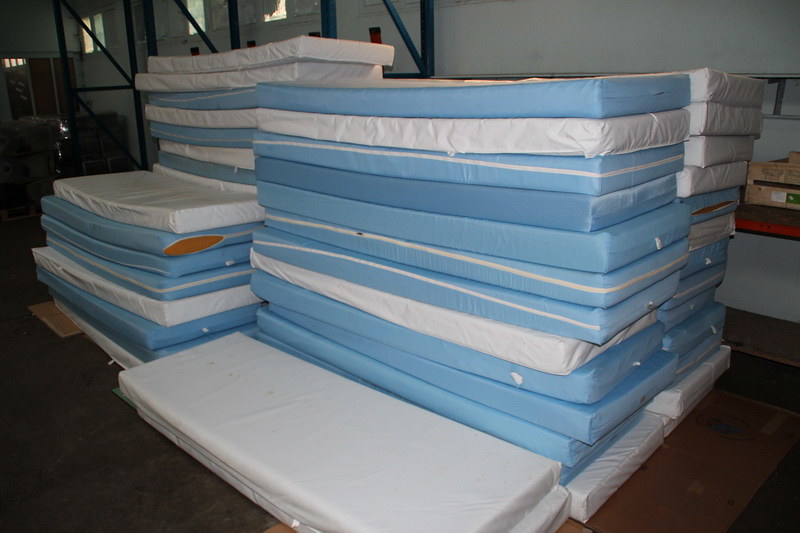This photograph depicts the interior of a warehouse with white walls and some metal ridging protruding from them. The floor appears to be wooden, contributing to the industrial aesthetic. Against the background, there is a mix of equipment including a small wooden box on the right side and a red bar, with light streaming through three windows. The primary focus is on several stacks of thin, rectangular mattresses or foam pads, each just a few inches thick. The mattresses are organized into five distinct stacks: two rows in the front and one in the back. In the front row, the left stack is composed of two mattresses piled atop each other, while the adjacent stacks each consist of 13 mattresses. Behind these, there is a stack of eight mattresses and another rising to about 14 or 15 mattresses tall. Each mattress is either covered with a white fitted sheet or enclosed in a blue sheet with a zipper around the center edge, suggesting some are plastic covers. This organized array of mattresses against the warehouse setting captures a scene that is both orderly and industrious.